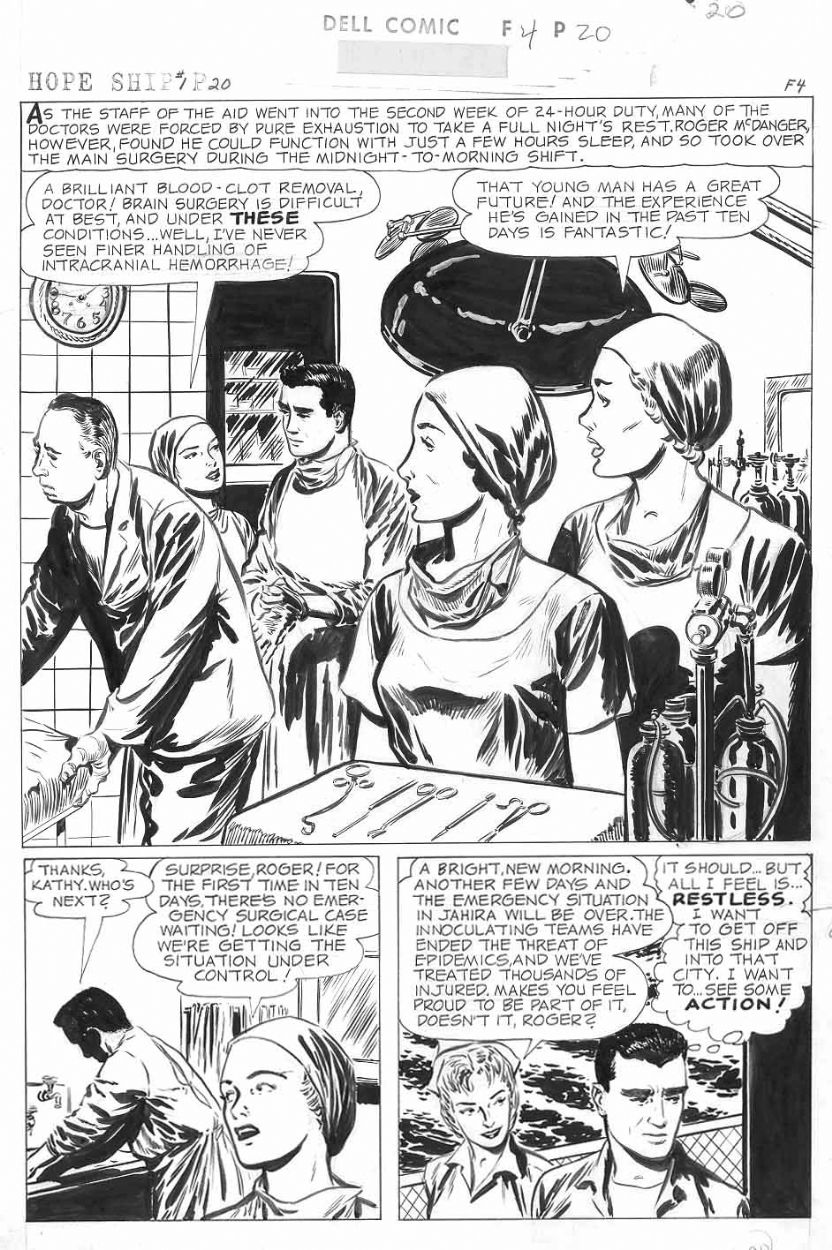This detailed black and white comic strip, "Hope Ship," is issue number 20 from Dell Comics. The comic opens with a dramatic scene showing medical personnel in a hospital environment. The top three-quarters of the page feature two nurses, one with her mouth open in visible concern, and a jet-black-haired doctor, Roger McDanger, scrubbing in for surgery. The accompanying text reveals the intense scenario: "As the staff of the aid went into the second week of the 24-hour duty, many of the doctors were forced by pure exhaustion to take a full night's rest. Roger McDanger, however, found he could function with just a few hours sleep and so took over the main surgery during the midnight to morning shift."

In this main panel, a nurse praises Dr. McDanger's skill, remarking on his brilliant blood clot removal and exceptional handling of brain surgery under daunting conditions. Another woman in the background notes his great potential and the invaluable experience he's gained over the past 10 days.

The bottom quarter of the page is divided into two panels. In the left panel, Roger is surprised to learn that for the first time in 10 days, no emergency surgical cases await. The nurse informs him, "Thanks, Kathy, who's next?" to which she responds, "Roger, for the first time in 10 days, there's no emergency surgical case waiting. It looks like we're getting the situation under control." The right panel depicts a brief dialogue about the progress they've made in the crisis area: "A bright new morning, another few days and the emergency situation in Tahira will be over. The inoculating teams have ended the threat of epidemics and have treated thousands of injured."

In a reflective moment, Roger's thought bubble reveals his inner conflict: "It should, but all I feel is restless. I want to get off this ship and into that city. I want to see some action."

The vintage artwork is striking in its detail, capturing the gravity and dedication of medical professionals in a crisis setting.